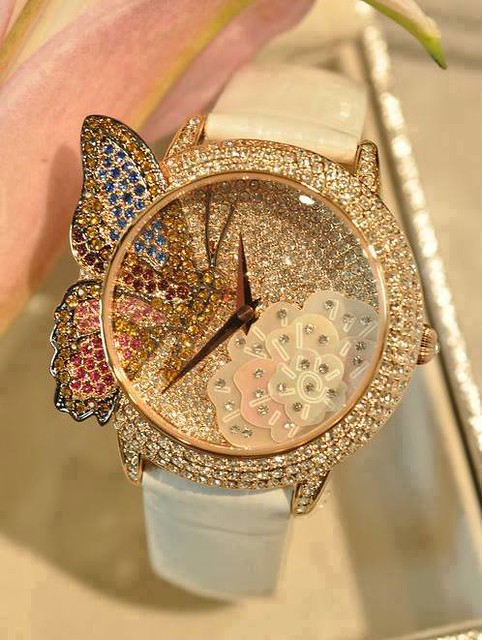In this captivating photograph, we see an exquisite ladies' watch displayed elegantly, most likely in a high-end store setting. The view is from above, showcasing the timepiece placed atop a luxurious display box. The watch features a pristine white leather band, complementing its opulent, round face. Intricately adorned, the right edge of the watch sparkles with a row of glistening diamonds. To the left, there's a plant accentuating the elegance of the overall presentation.

The standout feature of this watch is a shimmering butterfly embellished with an array of colorful jewels and countless diamonds, seemingly poised to land. This butterfly motif extends gracefully from the left side of the watch, adding a touch of whimsy and splendor. The watch face itself is a miniature garden, with delicate, diamond-studded flowers set against the dial, enhancing the theme of nature's beauty. Every inch of this spectacular timepiece is encrusted with dazzling diamonds, exuding an undeniable aura of luxury and sophistication. This meticulously crafted watch undoubtedly conveys a sense of unparalleled opulence and refinement.